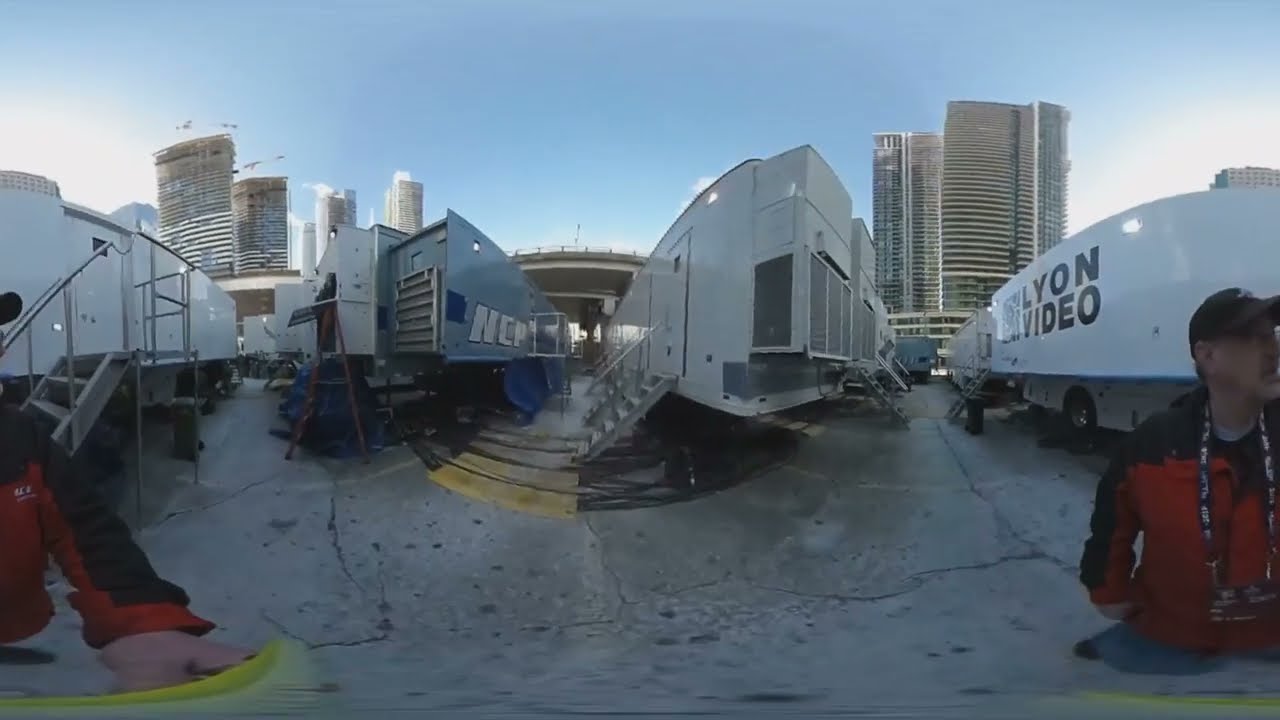This detailed image depicts an outdoor urban scene featuring tall buildings in the background against a clear blue sky. The foreground is dominated by several white portable trailers arranged on a large gray cement parking lot, with metal staircases providing access to their doors. A noticeable trailer on the right side is labeled "Lion Video" in black letters. 

In the right foreground, a white male wearing a red and black jacket with a dark-colored cap turns his head towards the camera. He sports a lanyard around his neck, though the text on it isn't discernible. Interestingly, the image appears stitched together, creating a warped effect where the same man’s left arm and torso are also visible on the far left side of the image.

To the left, another man stands nearby, also in a red and blue coat, possibly holding something yellow in his hand. Overhead, high-rise buildings loom, and in the far background, a bridge is subtly visible, emphasizing the urban setting. The day appears bright and clear, contributing to the vivid colors and overall clarity of the photograph.